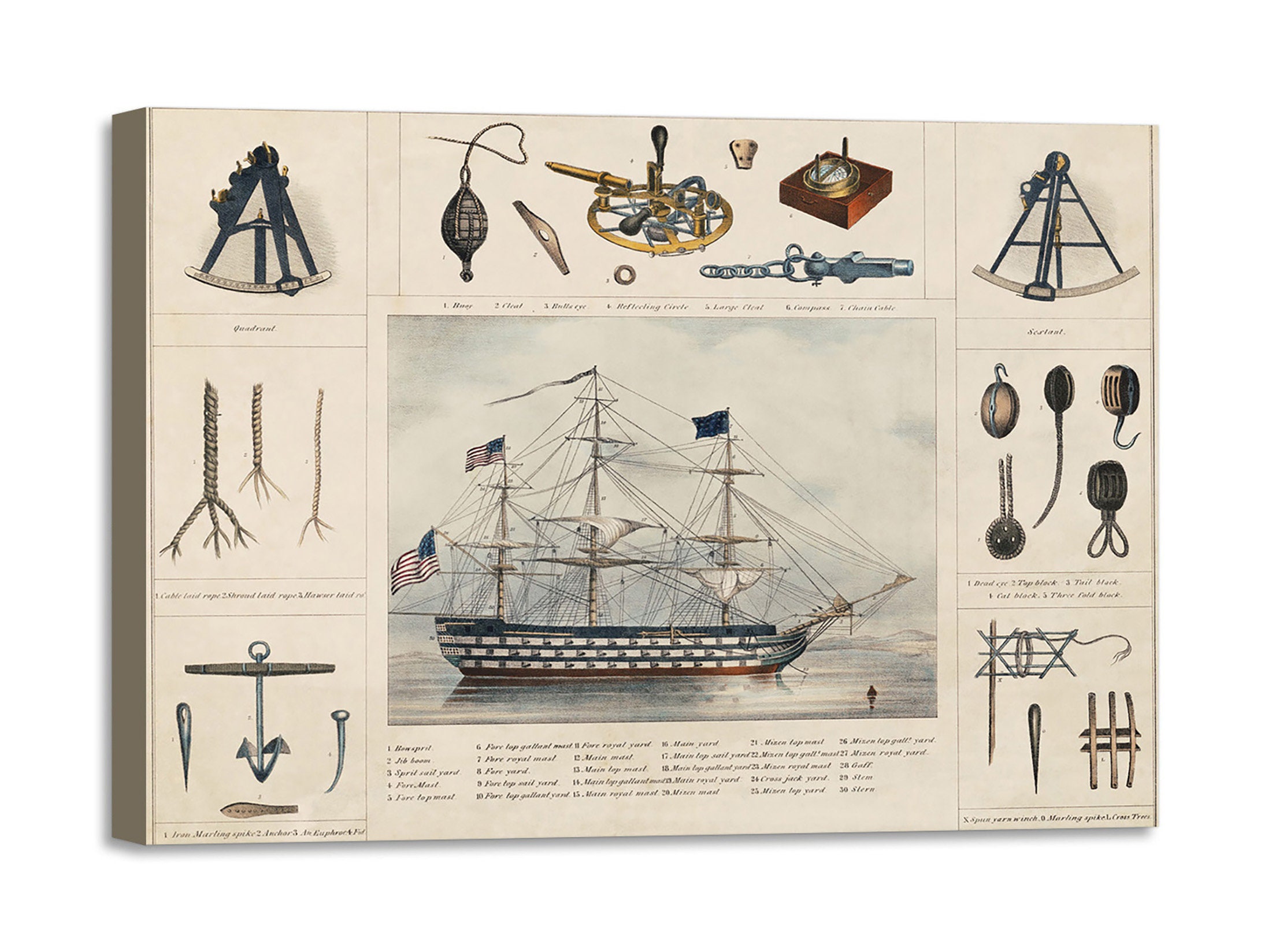This digital illustration is a detailed, color depiction of a large, historical sailing ship adorned with American flags. The central image features a majestic ship with three masts, each topped with a flag—two American flags and one black flag with stars. The hull of the ship is marked by a distinctive red stripe at the bottom, followed by alternating blue and white stripes. Surrounding this central image are various smaller illustrations of nautical equipment, including a compass, rope, anchor, sextants, tackle, and a marlin spike, offering a comprehensive view of seamanship tools. The top of the image features a rectangular section, while both the left and right sides contain three square insets, each showcasing different aspects of maritime interest, like detailed rope twists. Beneath the ship, there are six columns filled with text and numbered items, presumably listing and describing various ship components and their functionalities, indicating an informational purpose similar to a guide or educational sheet. The text below the ship is not fully legible but appears to extend the informational nature of the illustration, making it a rich resource for understanding the intricacies of sailing and seamanship.